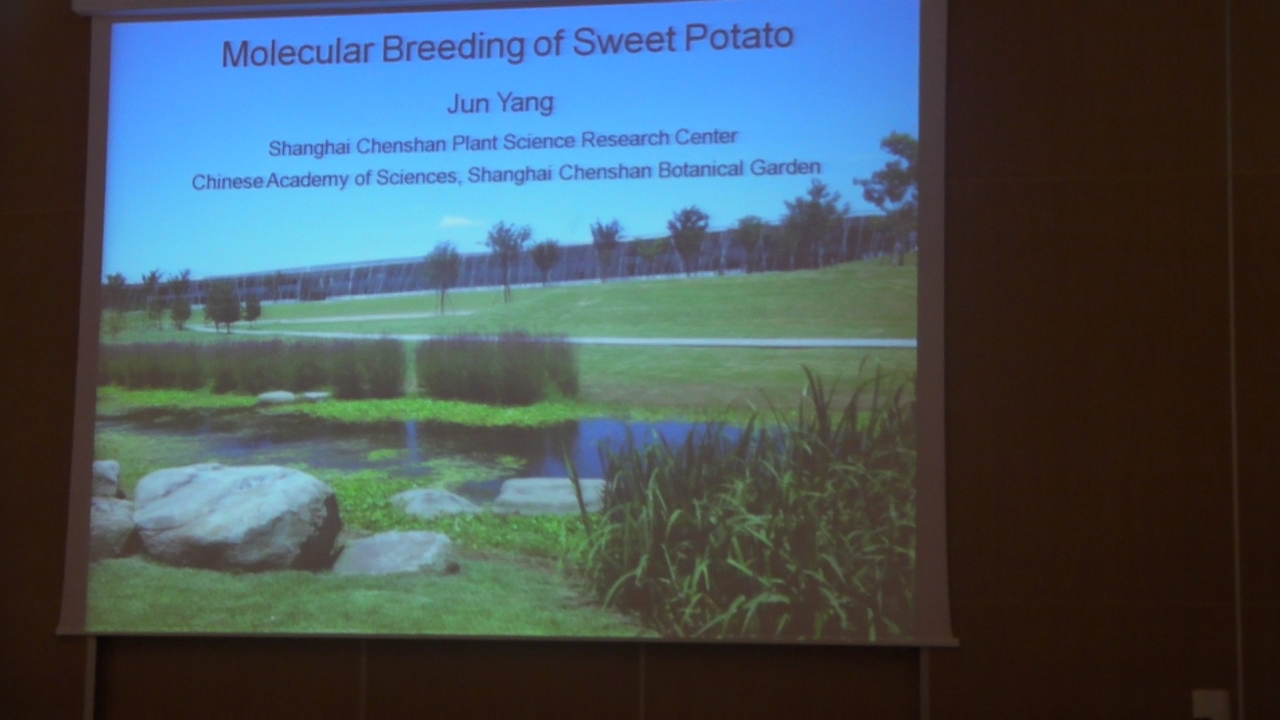In the auditorium, against a black velvet curtain, a projection screen displays a detailed field setting with a landscaped area under a clear blue sky. The screen, positioned toward the middle left, shows a composition of well-manicured grass, lush bushes, and a small creek surrounded by vegetation. Prominent larger rocks lie in the foreground on the left, while a concrete pathway extends into the grassy field. Taller trees with green leaves form the backdrop. Overlaying the image is black text that reads, "Molecular Breeding of Sweet Potato," followed by "Jun Yang," and "Shanghai Chenshin Plant Science Research Center, Chinese Academy of Sciences, Shanghai Chenshin Botanical Garden."